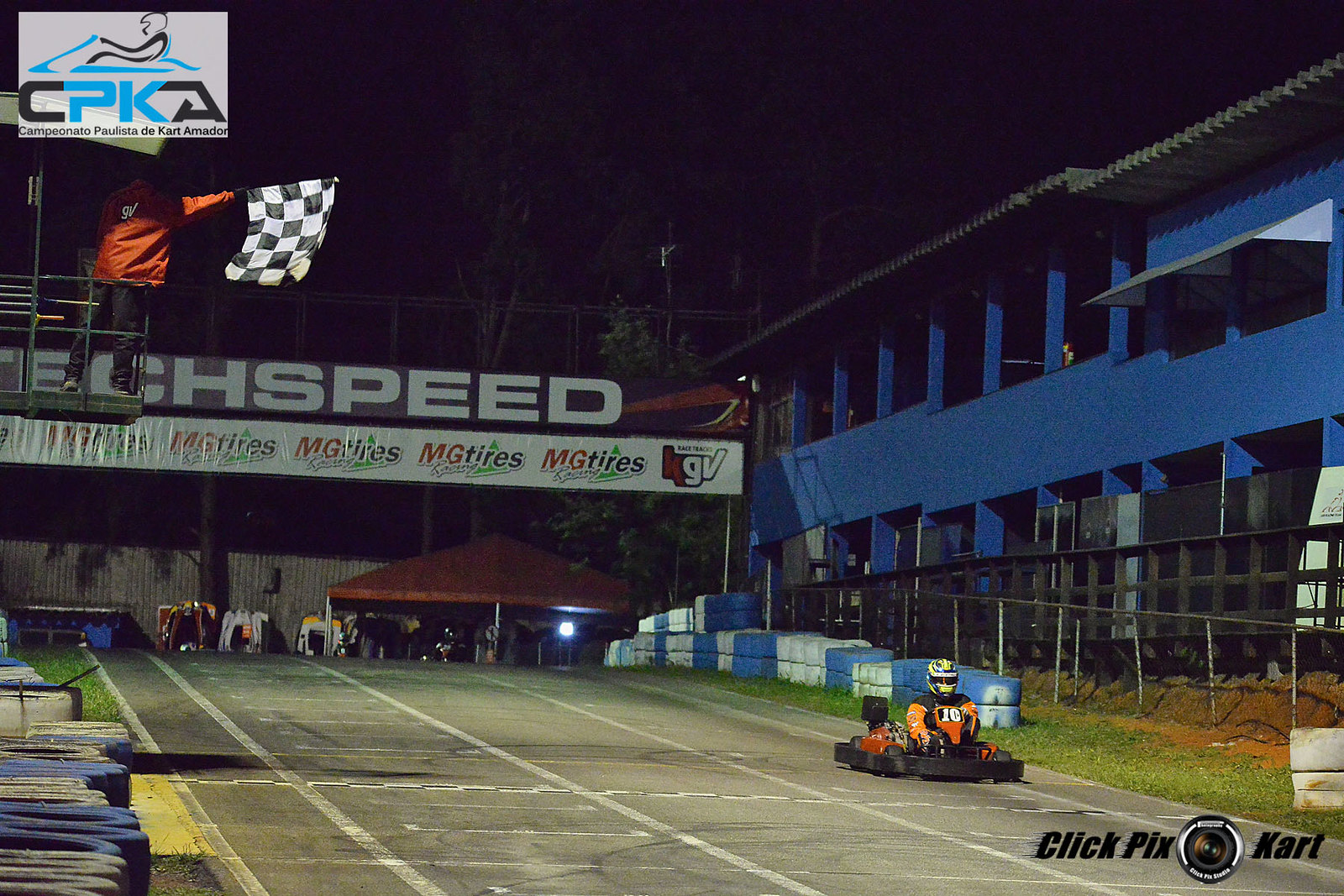The image captures a detailed scene of a go-kart track bustling with activity. In the upper left-hand corner, the CPKA logo prominently displays the letters 'P' and 'K' in blue, while 'C' and 'A' are in black, creatively forming part of a sketched go-kart with a black-outlined driver. Standing below the logo, a man in a red jacket holds a checkered black and white Czech flag, facing away from the camera, indicating the start or end of a race. Behind him, the banner with the black 'TechSpeed' logo and another advertising MG Tires are clearly visible.

The go-kart track itself is a faded gray color with white lines demarcating three lanes, hinting at its capacity for multiple racers. In the upper right-hand corner, a racer in an orange and black suit is ready to speed off in a go-kart, possibly indicating the start of a trial run or the race’s finishing stretch. Above this racer, the words "ClickPixKart" are displayed, with a blue building featuring open windows forming the backdrop. The entire scene implies an organized, competitive environment at a go-kart racing venue.